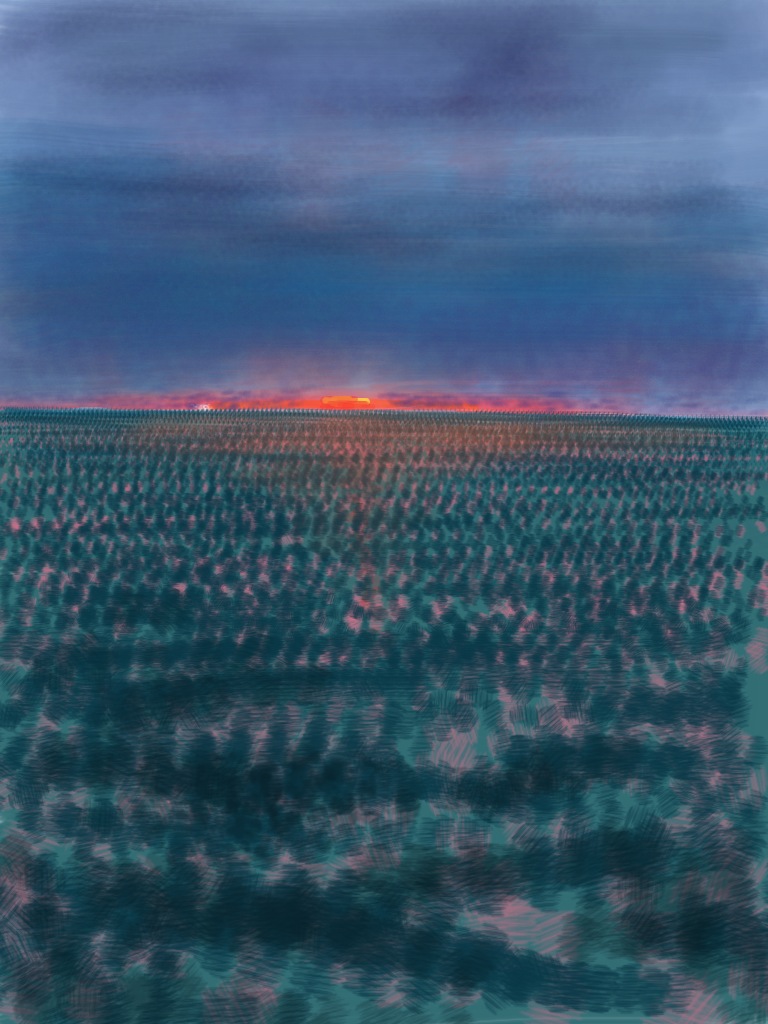The artwork appears to be a mixed-media painting, likely acrylic and possibly incorporating watercolor techniques, capturing a serene twilight scene. In the upper part of the image, the sky features a blend of dark blue and periwinkle hues with tinges of purple, evoking a misty, cloudy evening. The horizon glows with vivid oranges and magentas, indicating either a setting or rising sun that casts radiant light across the scene, though the sun itself is not distinctly visible. Between the glowing horizon and the vivid sky lies an expansive ocean, occupying roughly two-thirds of the canvas. This ocean is portrayed with variegated shades of blue, green, and subtle hints of pink, giving a textured and somewhat abstract appearance with soft white highlights suggesting waves or reflections. The overall composition is soft and blurred, creating an ethereal, almost dreamlike atmosphere. The scene’s distinctive lack of harsh edges and the melding of colors emphasize the tranquil and hazy quality of this captivating sunset over the ocean.